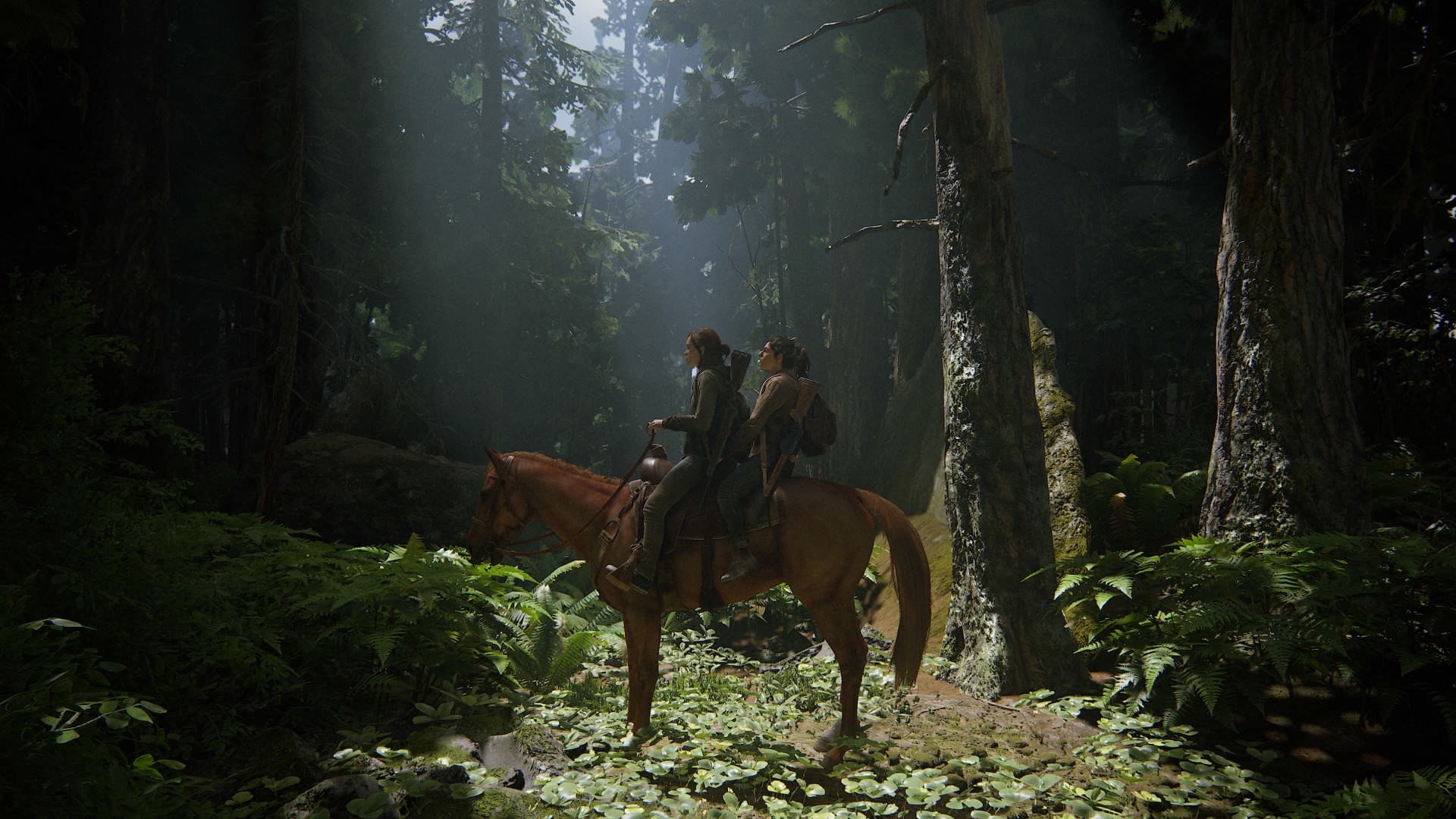In this detailed digital rendering set in a forest, sunlight streams down between the dark trees, illuminating a small clearing. In the center bottom of the image stands a brown horse, appearing red in the light, outfitted with a saddle and bridle. Atop the horse, two women with dark hair pulled back in ponytails are seated. The first rider, wearing a jacket, long pants, boots, and a rifle attached to her back, holds the reins. The second rider sits behind, holding the first, with a backpack on her back and a gun as well. Surrounding them, tree trunks bathed in sunlight contrast against the dark green leaves and occasional glimpses of sky, while light green plants cover the forest floor beneath the horse. Despite being a digital artwork with elements seemingly superimposed, the scene vividly captures the tranquil, sun-dappled forest setting in daylight.